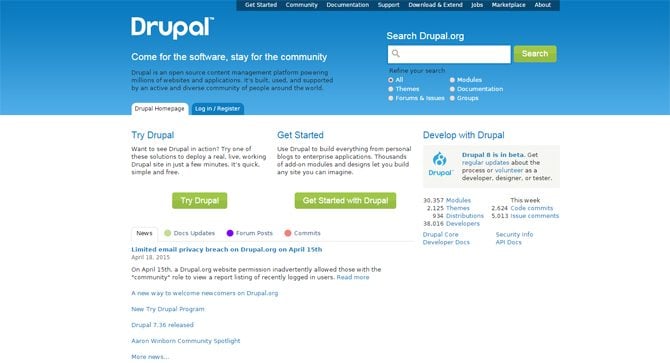**Detailed Caption:**

The webpage features a dark blue header at the top with multiple clickable buttons, including "Get Started," "Community," "Documentation," and "Support." Further options such as "Download and Extend," "Jobs," "Marketplace," and "About" are also available. On the left-hand side, the word "Drupal" is prominently displayed multiple times in large, bold white text. Beneath this, in smaller bold white text, the phrase "Come for the software, stay for the community" is featured.

A rectangular search bar is located on the right-hand side, containing a gray magnifying glass icon and the phrase "Search Drupal.org" above it. To the right of this search bar is a green clickable button with bold white text that reads "Search."

Below this section are several clickable tabs, with "All" being the currently selected tab. Additional tabs include "Themes," "Forums," "Issues," "Modules," "Documentation," and "Groups." 

The webpage further reads: "Try Drupal" in bold blue text, followed by a black text line that says "Want to see Drupal in action? Try one of these solutions to deploy a real live working Drupal site in just a few minutes. It's quick, simple, and free." Below this, there is another line in bold blue text that urges users to "Get started."

An informational section follows, explaining how to "Use Drupal to build everything from personal blogs to enterprise applications" and highlighting that thousands of add-on modules and designs are available to create any site imaginable. 

The section "Develop Drupal" is displayed in blue, accompanied by the Drupal icon, which is a blue teardrop shape with a white "D" in the center. Underneath this icon, "Drupal" is clearly labeled.

Finally, there are two prominent green clickable buttons on the left-hand side: one under "Try Drupal" and another under "Get Started." Both buttons feature bold white text, encouraging users to engage with Drupal's features and services.